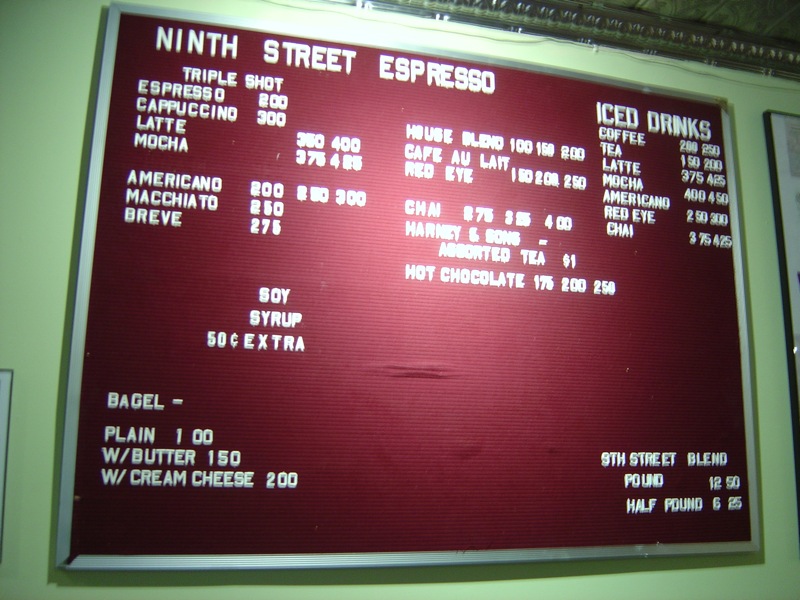**Caption:**

A detailed glimpse of the vibrant menu at 9th Street Espresso, a cozy coffee shop with a modern aesthetic. The menu, mounted on a wall painted in a refreshing lime green, features a chic chrome trim and a striking reddish background. The white font clearly categorizes a variety of beverages and offerings.

**Triple Shot Category:** 
- Espresso
- Cappuccino
- Latte
- Mocha
- Americano
- Macchiato
- Breve

Options include soy syrup for an additional 50 cents.

**Bagels:** 
- Plain with butter
- With cream cheese

**Iced Drinks Category:** 
- Iced Coffee
- Iced Tea
- Iced Latte
- Iced Mocha
- Iced Americano
- Iced Red Eye
- Iced Chai

**Hot Beverages:** 
- House Blend
- Café au Lait
- Red Eye
- Chai
- Marnie and Sons Assorted Tea
- Hot Chocolate

Additionally, patrons can purchase the 9th Street Blend coffee by the pound or half-pound. Each item on the menu is accompanied by its respective price, ensuring clarity and convenience for customers.